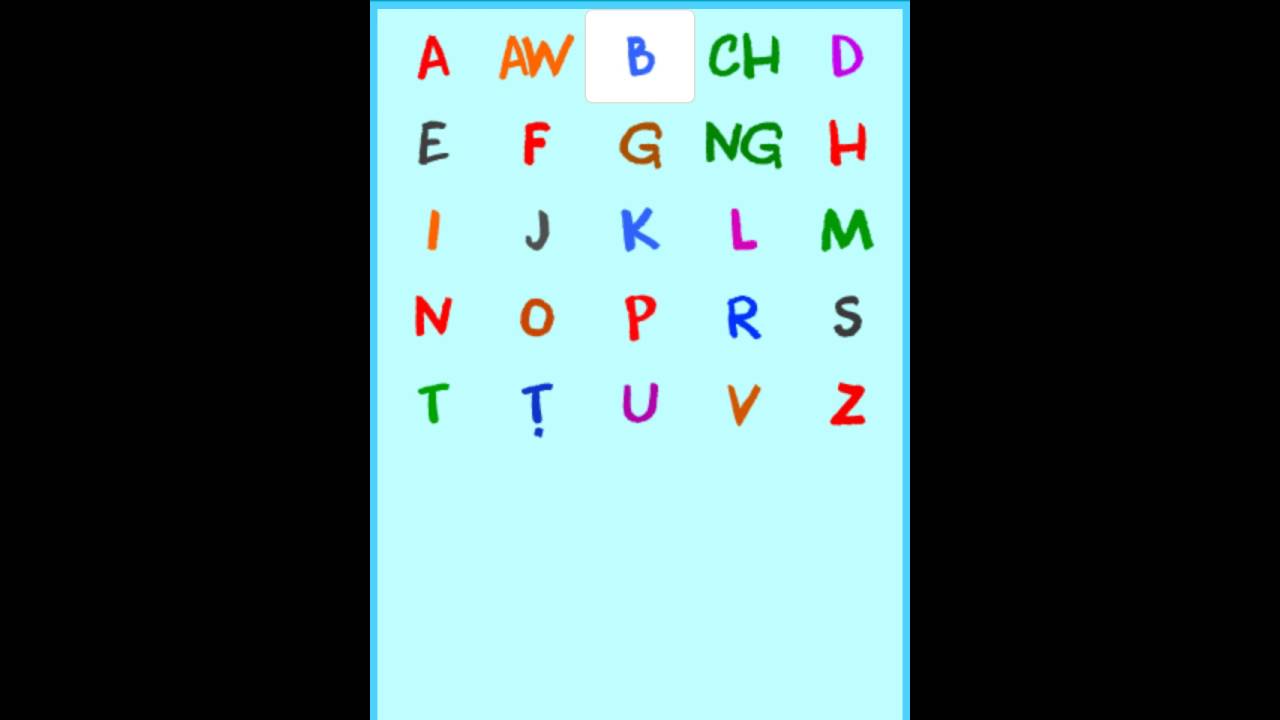The image features a vertical, light blue rectangle as the main focal point. Inside this rectangle, five rows of letters are listed, each varying in color. At the very top of the rectangle, the letter "A" is displayed, followed by an orange "AW." The first row then includes the letter "B" in blue, set against a white square, "CH" in green, and finally "D" in purple. 

The second row consists of the letters "E" in black, "F" in red, "G" in brown, "NG" in green, and "H" in red. The third row presents "I" in orange, "J" in black, "K" in blue, "L" in purple, and "M" in green. 

In the fourth row, "N" is shown in red, "O" in brown, "P" in red, "R" in blue, and "S" in black. The fifth and final row includes "T" in green, "T" with a small dot underneath in blue, "U" in purple, "V" in brown, and "Z" in red.

Surrounding this blue box, there is a long black rectangle on the left side, and another long black rectangle on the right side.